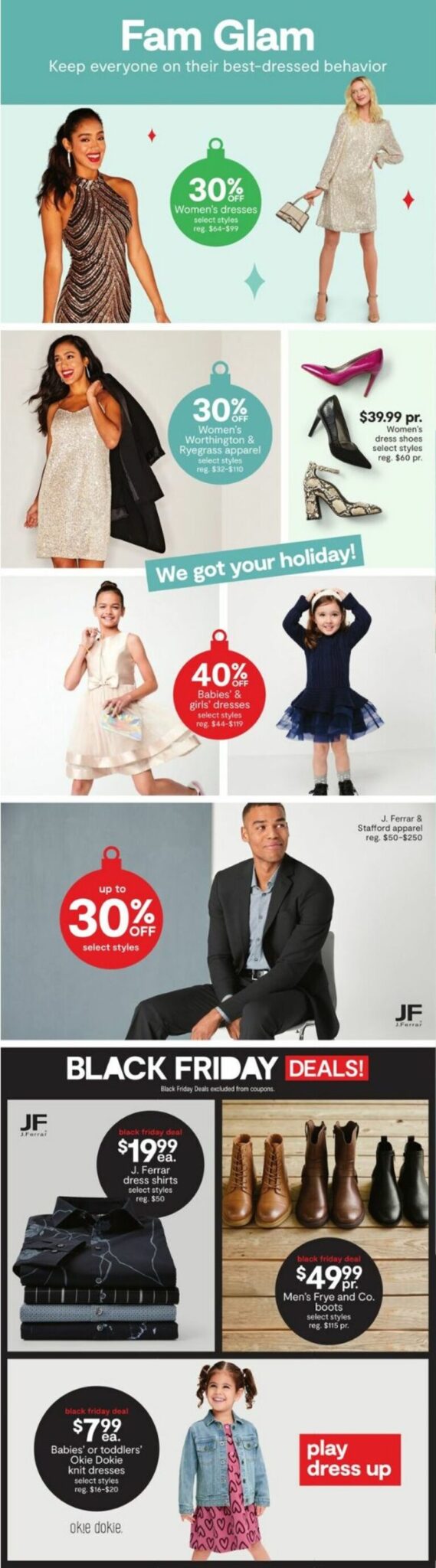This advertisement is composed of several distinct sections, visually outlined to entice the viewer. At the top of the ad, the bold letters spell out "FAMiliary," with "Glam" immediately following, hinting at a family-oriented yet fashionable theme. The tagline below reads, "Keep everyone on their best-dressed behavior," setting a stylish and aspirational tone.

The left section of the ad features a woman with shoulder-length black hair, radiant with a smile. She is elegantly dressed in a striking bronze and black dress. Centrally placed text announces "30% off Women’s Dresses," specifying that select styles ranging from $64 to $99 are included in the offer.

To the right, another image showcases a different woman adorned in a long-sleeved white dress. She complements her attire with heels and carries a stylish bag in her right hand. Her blonde hair cascades down, adding to her sophisticated appearance.

The section below continues with an image on the left of yet another woman, this time with black hair, dressed in a chic white dress. She effortlessly holds a black coat over her left shoulder, exuding a casual but polished look. The text on the right reinforces the promotional message with "30% off."

Overall, this advertisement is visually compelling with its array of stylishly dressed women, emphasizing a glamorous yet accessible fashion trend for all.